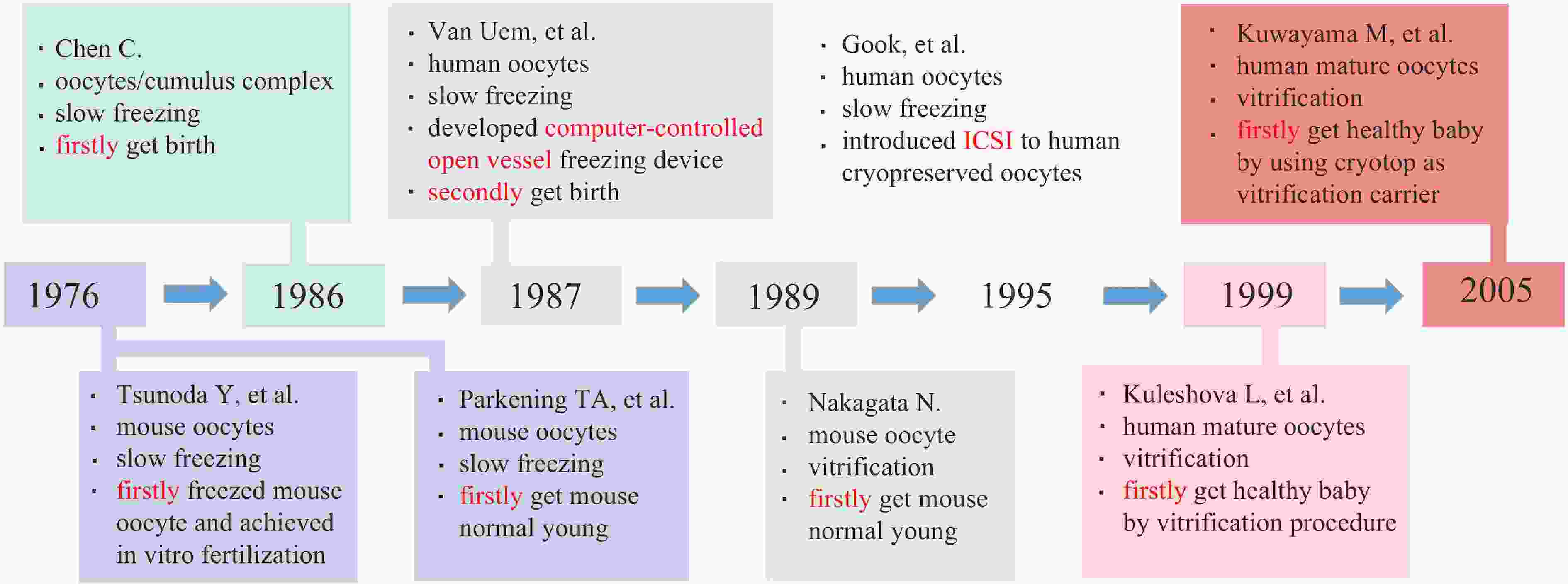The diagram illustrates a detailed timeline of scientific milestones from 1976 to 2005. Encased in a horizontally rectangular layout, the timeline is divided into three rows with color-coded boxes containing text. The middle row displays the key years: 1976, 1986, 1987, 1989, 1995, 1999, and 2005, connected by blue, gray, light gray, and brown arrows indicating progression.

At the top row, linked to 1986, are four bullets: Chen Xi, Uppsity’s first last cumulus complex, slow freezing, and "firstly get birth." Meanwhile, the bottom row branches out from 1999 with four bullet points: Kulasava L., et al., human mature Uppsity, vitrification, and "firstly get healthy baby by vitrification procedure."

The detailed annotations for each year provide important contributions:

1. **1976**: Two blue boxes highlight significant achievements:
   - **Tsunoda Y. et al.**: Describes the slow freezing of Mao’s old sites, marking the first successful in vitro fertilization.
   - **Parkinian T.A. et al.**: Notes the first successful freezing of Mao’s old sites resulting in normal young Mao’s.

2. **1986**: A blue box points to this year, with annotations indicating vital advancements.

3. **1987**: A gray box marks further progress.

4. **1989**: Linked by another gray box, indicating continuous developments.

5. **1995**: Indicated by a light gray box pointing downwards.

6. **1999**: A pink box at the bottom row lists contributions such as:
   - **Kulasava L. et al.**, human mature Uppsity, and vitrification leading to the first healthy baby by this procedure.

7. **2005**: A brown box notes a breakthrough:
    - **Kua Yama M.**: Highlights the use of cryotop as a vitrification carrier for human mature old sites, achieving the first healthy cryotop vitrified baby.

Overall, the diagram clearly marks key achievements in reproductive science, connected through a series of arrows and color-coded boxes, making it a comprehensive guide to the advances over three decades.